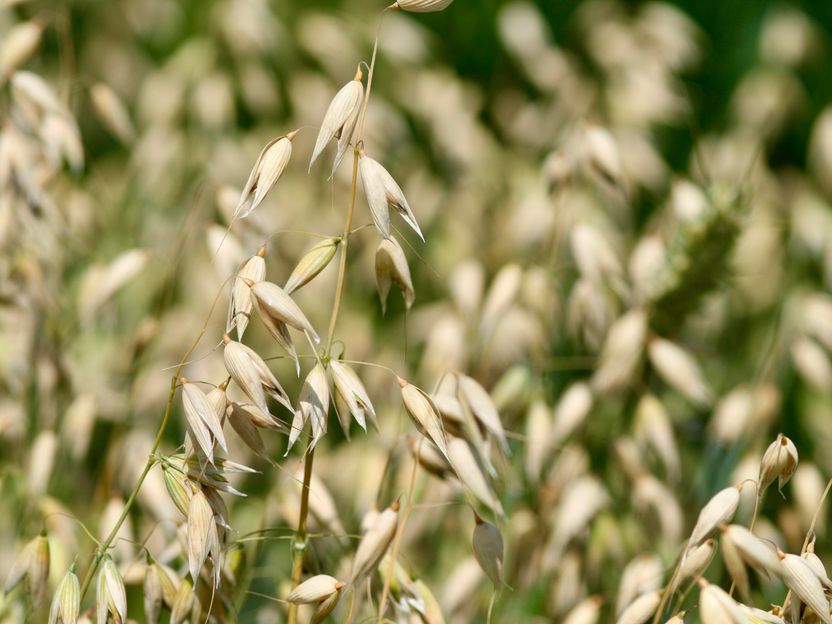The image is a close-up shot of a flower against a blurred background that hints at a large field of similar flowers. Dominated by a tan and green palette, the photo features a tall, slender tan and green stem situated slightly to the left. This main stem is adorned with thin, side stems, each ending with drooping, oval-shaped petals that are tan-colored and elongated. The petals appear either partially open or already wilted, with pointed tips suggesting a past prime. The background, suffused with a strong bokeh effect, reveals more of these flowers and hints of green foliage that indicate a sunny field. The overall atmosphere conveys a natural, outdoor setting, possibly a field of crops, underlining the seasonal cycle of bloom and decay.